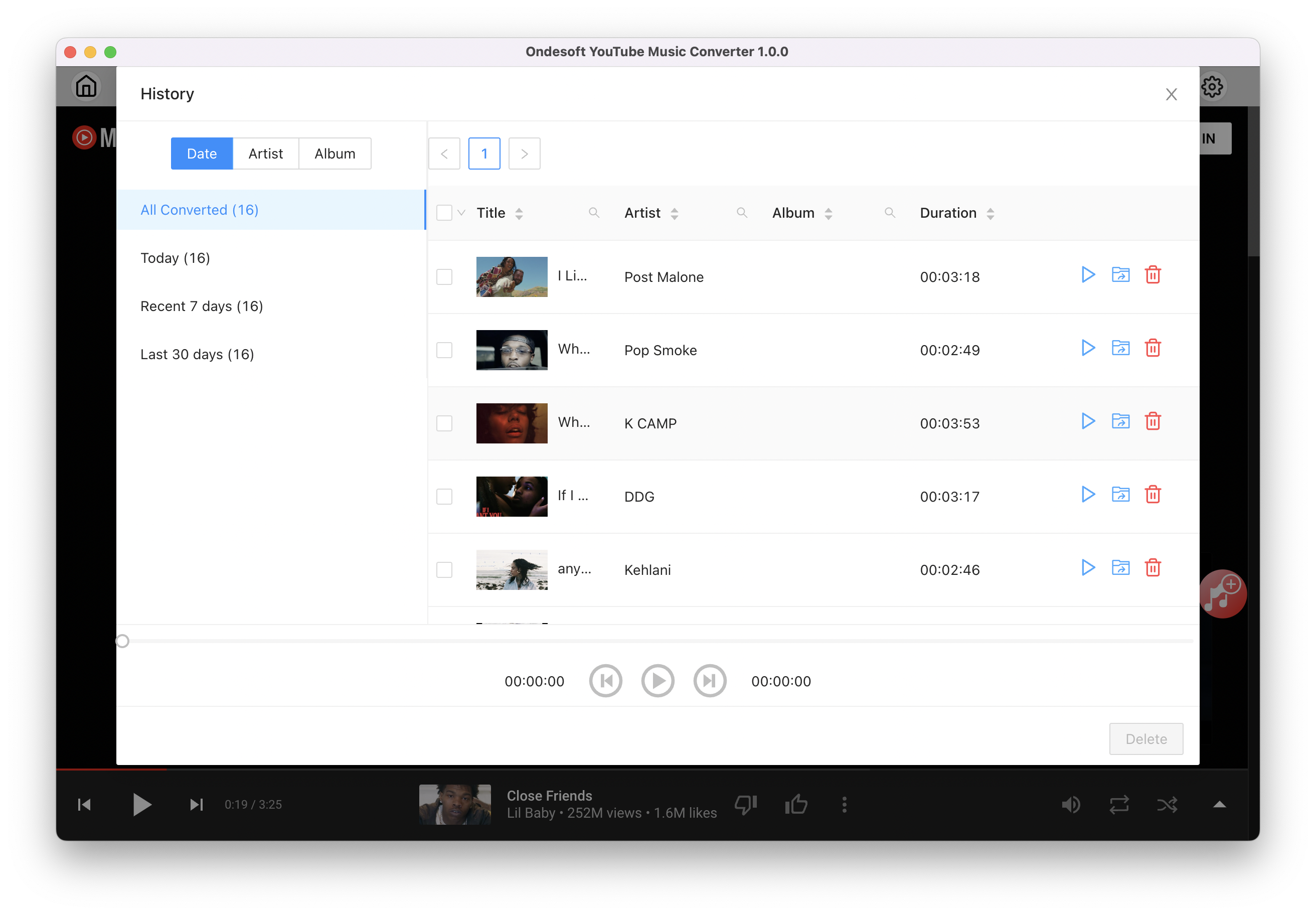This image features an OND Soft YouTube Music Converter interface. At the top center, the title "OND ES OFT YouTube Music Converter 1.0.0" is prominently displayed. Overlaying a distinctive YouTube-themed background, there is a white pop-up window labeled "History." In the upper left corner, the window features a series of three dot indicators colored red, yellow, and green. On the left side of the pop-up window, three buttons labeled "Date," "Artist," and "Album" are aligned side-by-side. Below these buttons lies a vertical menu with categories including "All Converted: 16," "Today: 16," "Recent seven days: 16," and "Last 30 days: 16." To the right of this menu, a list displays various musical artists, including Post Malone, Pop Smoke, K Camp, DTG, and Kehlani.